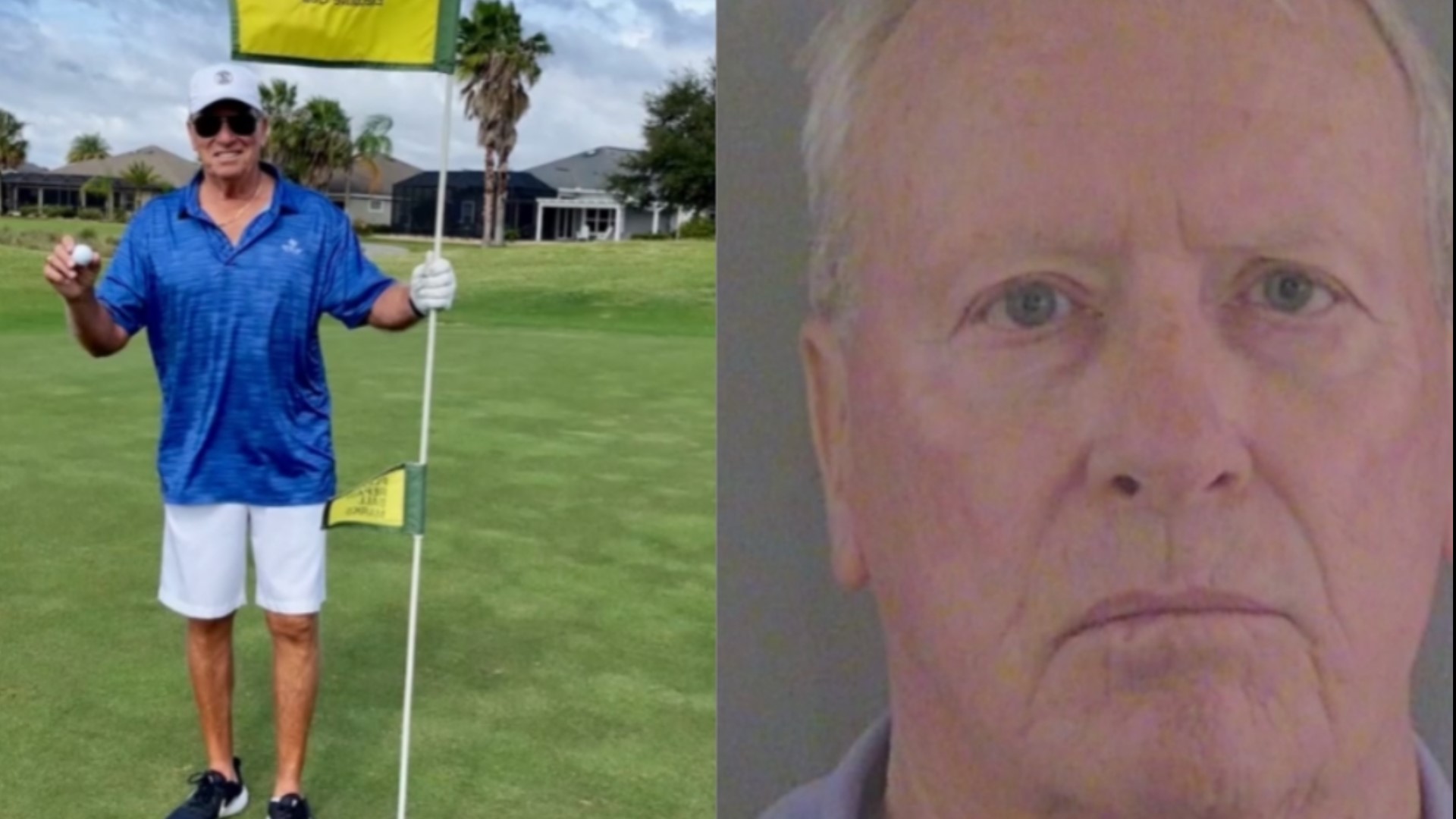This rectangular image juxtaposes two photos of presumably the same older white man. On the right, a close-up, mug shot-like photograph captures the man’s stern and slightly frowning expression, with short gray hair and a gray background. Although he sports a collared shirt, only the neckline is visible. On the left, the man appears in a contrasting setting: a vibrant, manicured golf course. Here, he is joyfully smiling, clad in a white baseball cap, black sunglasses, a blue short-sleeve polo shirt, white shorts, and black tennis shoes. He holds a golf ball in one hand and a flagstick topped with a green and yellow flag in the other. The backdrop includes a panoramic view of palm trees, houses, mountains, and blue sky, accentuating the outdoor leisure scene.